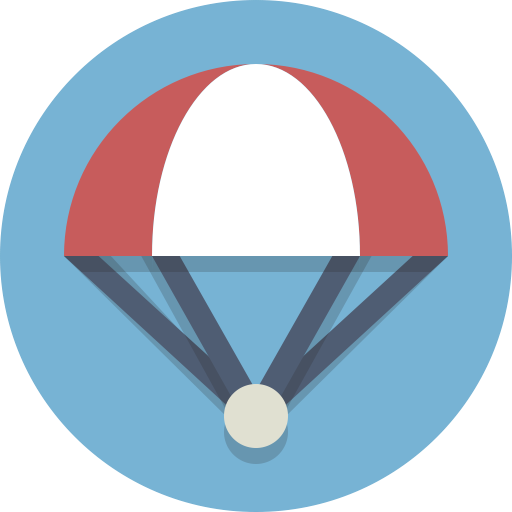The image features a centrally positioned, computer-generated icon resembling a parachute against a plain white backdrop. Dominating the scene is a large, dull blue circle, within which lies a red and white alternating semi-circular shape evocative of a parachute canopy or umbrella top. This semi-circle, with a coherent pattern, forms the upper portion of the icon. The design includes four thick black lines—two descending from the right and two from the left—each converging at a small, central white circle near the bottom of the blue area. Notably, the depiction is enhanced by subtle shadows cast by the lines and the small white circle, adding depth. This minimalist composition is purely graphical, devoid of any textual elements or external references.